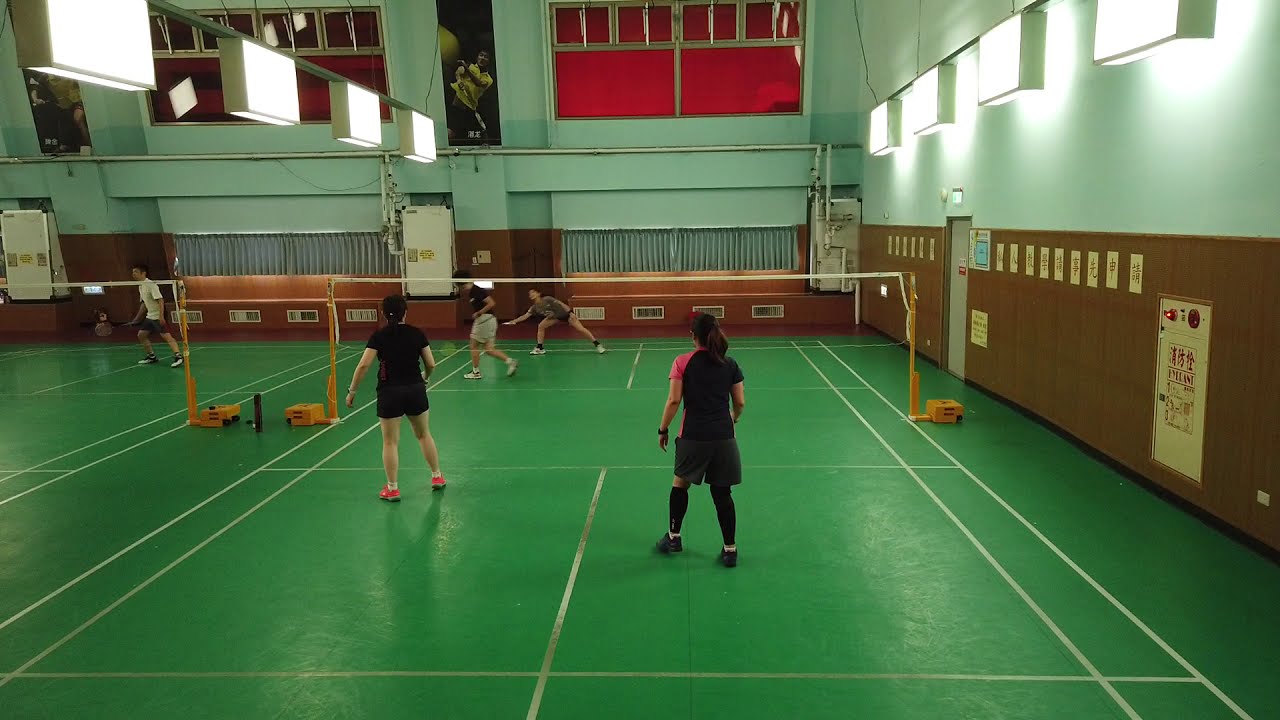Inside a spacious gymnasium with high, rectangular lights overhead, two badminton courts are prominently featured. The upper portion of the walls is painted a light green, contrasting with the brown lower half, while red shades or drapes adorn the upper-level windows. The floor of the courts is a rich green color, creating a vibrant backdrop for the activities within.

On the court to the right, two women in darker uniforms stand closest to the camera, one in shorts and the other in leggings. Across the net, another pair of players—a woman in a black top and a man in a gray top—are in mid-game action. In the background to the right, a man is reaching down as if retrieving a ball. Further to the left, another partially visible court shows a player in a white T-shirt engaged in play.

Additional details include white structures along the back wall, possibly containers or equipment, alongside some wall adornments featuring text, likely in an East Asian script, and pictures. The main colors in the image are green, red, brown, and white, contributing to the gym's lively and dynamic atmosphere.